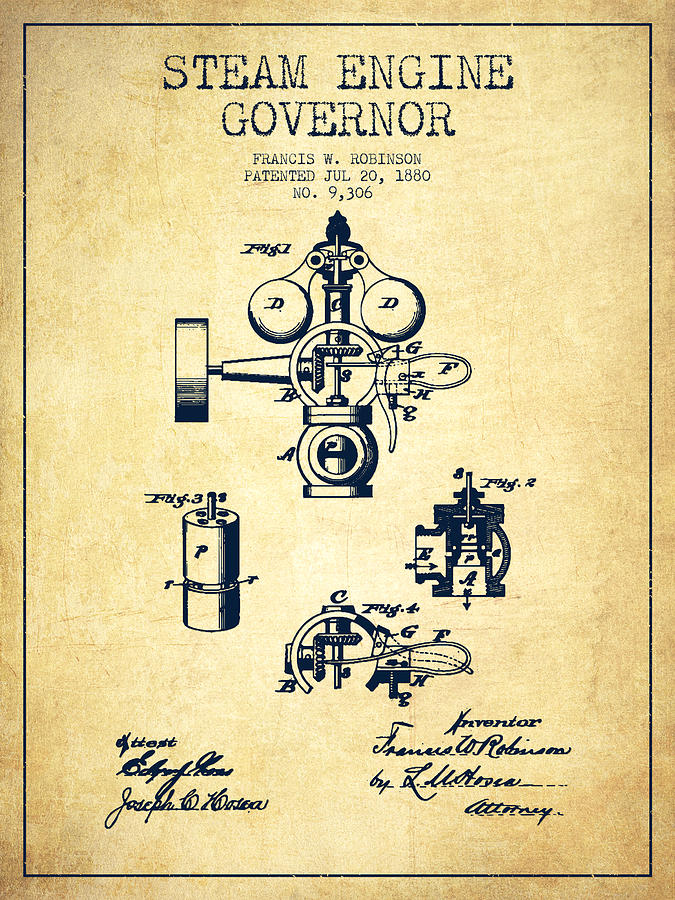This image seems to be a historic page, possibly extracted from an old book or patent application, dating back to July 20, 1880, as indicated by the typography. The page has an aged, yellowed appearance, akin to faded newsprint, and is framed by a thin black outline. Centered at the top in black typewriter-style font is the title "Steam Engine Governor," followed by the name "Francis W. Robinson." Below that, it states "patented July 20, 1880," along with the designation "No. 9,306."

The heart of the page showcases detailed pen-and-ink illustrations, portraying four distinct components of the steam engine governor, each labeled alphabetically from A to G. These technical drawings are precise and neatly arranged, highlighting various parts, including a cylinder and a mechanism that likely influences the governor's behavior.

At the bottom of the page, several cursive signatures appear on both the left and right sides, with three signatures on each side. One signature identifies the inventor, "Francis W. Robinson," and another, although partly illegible, is accompanied by the word "Attorney."

Overall, this document exemplifies an early patent application format, complete with formal notations, meticulous diagrams, and multiple endorsements, capturing a meaningful snapshot of 19th-century engineering documentation.